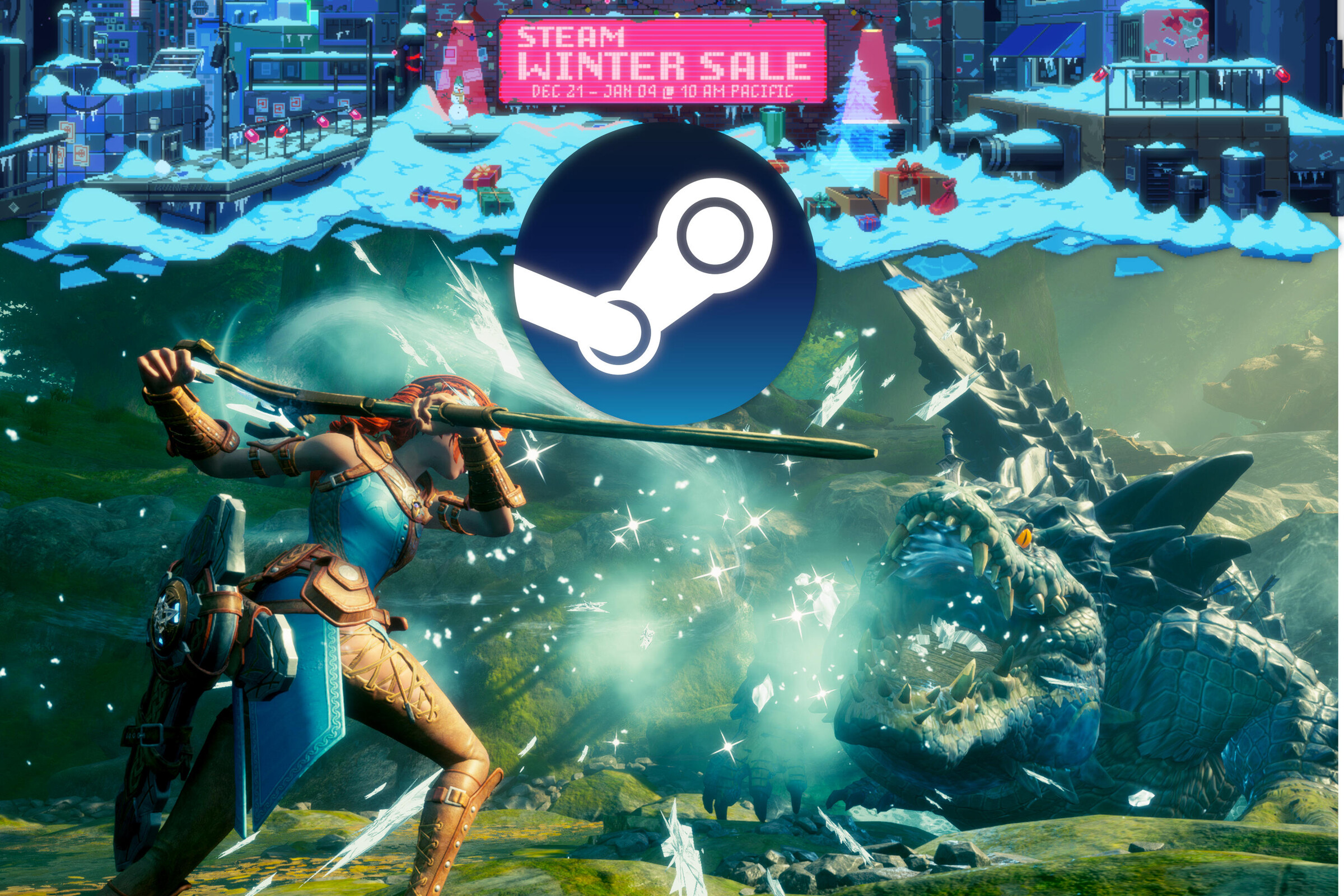This detailed illustration appears to be a promotional piece from a science fiction comic or video game, likely advertising a Steam Winter Sale. Dominating the foreground is a fierce, red-haired female warrior in blue armor, wielding a long saber and engaging in battle with a monstrous alligator-like creature, reminiscent of those in Godzilla movies. Her outfit is accented with gold and features a tool belt hanging from her waist. This intense battle scene unfolds against the surreal backdrop of a snow-covered urban landscape decorated with holographic Christmas elements like a tree and a snowman, alongside gift-wrapped presents scattered about. At the top center of the illustration, digital text announces the Steam Winter Sale, running from December 21st to January 4th at 10am Pacific, with a blue circular logo resembling a gear prominently displayed just below the festive announcement.